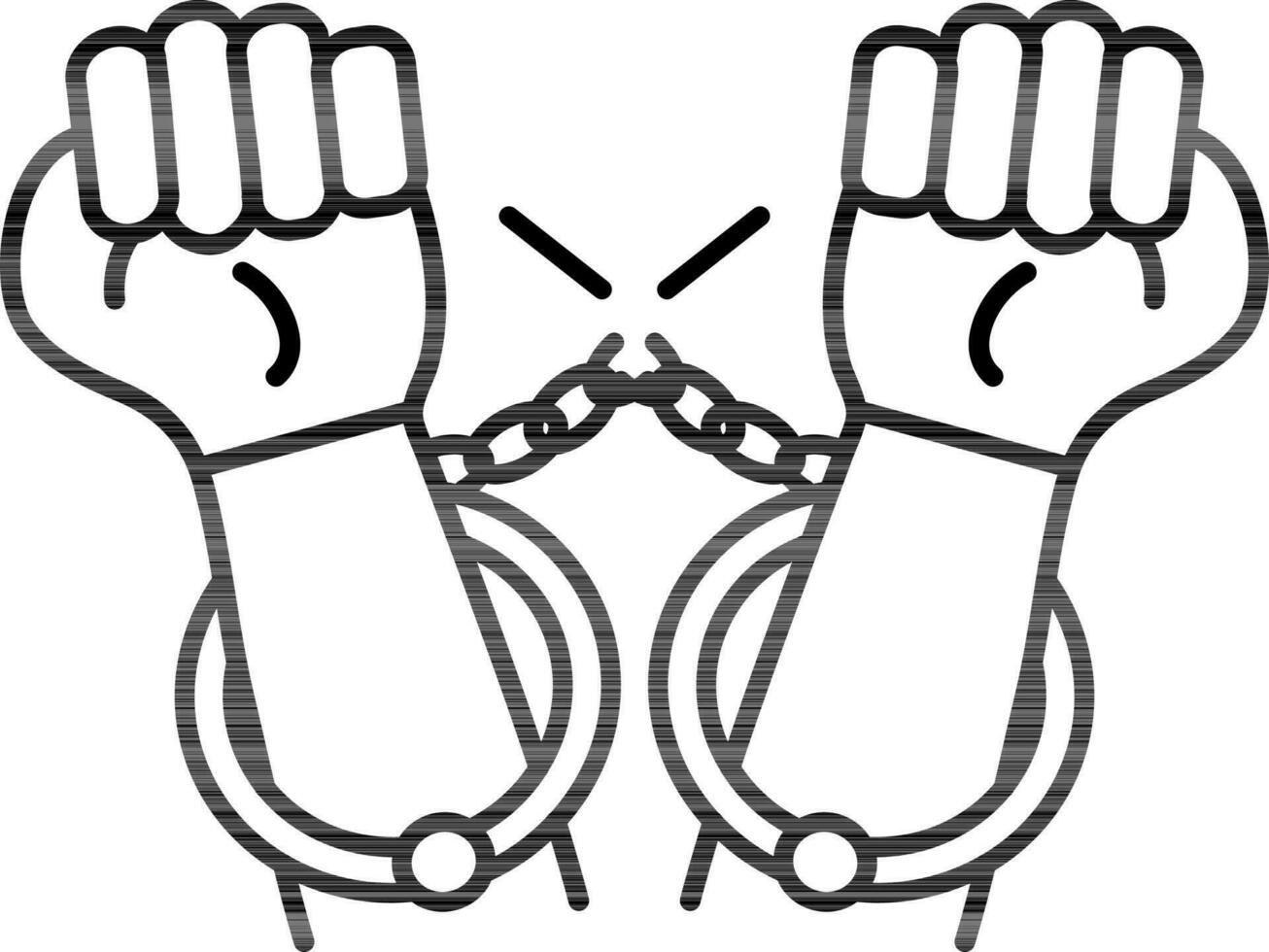This minimalist black-and-white drawing vividly captures the striking moment of liberation. Depicting only the forearms and fists of two hands, one left and one right, the image reveals the wrists bound by handcuffs. Despite the clasps still encircling each wrist, the chain connecting them has been snapped and is in the process of breaking apart, symbolizing a powerful act of breaking free. The hands, clenched into fists, are pulling away from each other, emphasizing the struggle and resistance. The graphic artistry combines clear, bold lines with some faded detailing, portraying the dynamic action of freedom as if the person is actively liberating themselves from the restraints.